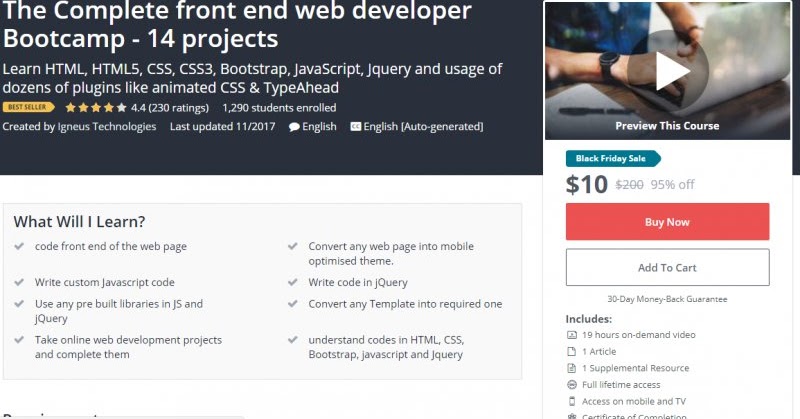**Image Description:**

On a black background occupying about two-thirds of the image starting from the left corner and extending halfway down, the top left corner prominently features bold white text that reads "The Complete Front-End Web Developer." Below this title, the text "Bootcamp - 14 Classes" is displayed. Further down, in smaller white lettering, additional information is provided on two lines. Positioned below this text is a gray tab with black text that says "Bestseller." 

Right beneath the bestseller tab, there are four yellow stars and one gray star, indicating a 4.4 rating out of 5 from 230 reviews. Additionally, it mentions that 1,290 students are currently enrolled. Following this, more details are offered in smaller white text, stating the course was created by [Author's Name] and noting the last update, with instruction in English.

To the right of this information, there is a small profile picture representing a video thumbnail, showing a man's hands typing on a laptop with a play button overlay in the center.

Across the image's bottom, in white text, it says "Preview This Course." Encircling this text is a thin white border extending to the bottom edge of the image. Positioned within this border, there's a teal tab stating "Black Friday Sale" in white text. Beneath this, bold black text prominently displays "$10," and a smaller "$200" with a strikethrough, indicating a 95% discount. Adjacent to this price tag is a red tab with white text saying "Buy Now," followed by a white tab with a black border that says "Add to Cart" in black text. Additionally, it mentions a "30-Day Money-Back Guarantee" below these options.

Towards the lower left corner, bold text reads "Inclusions," followed by a list of six items detailing what is included in the course. Above this list, smaller text in the top left corner says "What Will I Learn," followed by four checkmarks with corresponding information to the right. On the right side, there are an additional four checkmarks with lines of information beside them, elaborating on the learnings offered by the course.